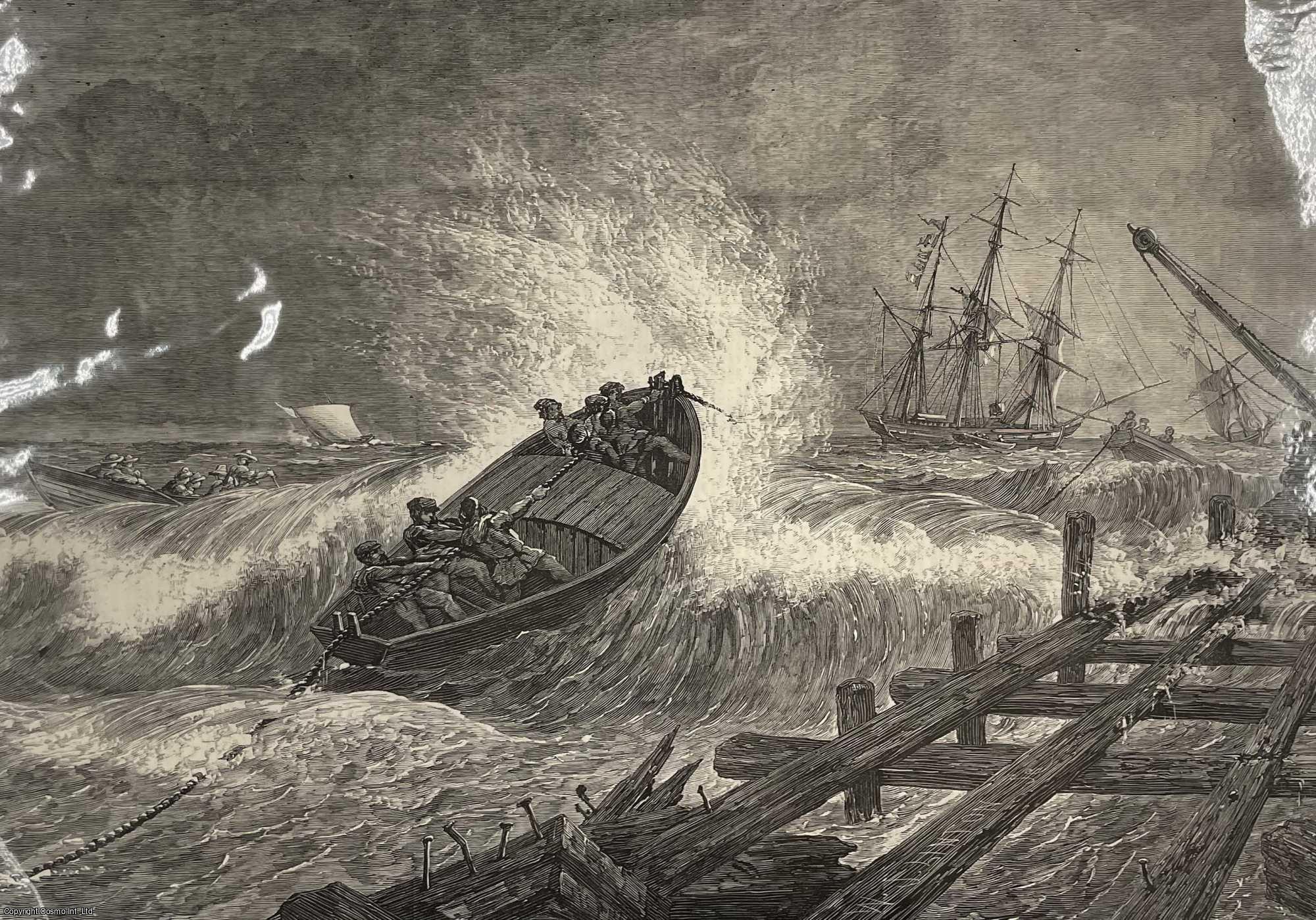This is a detailed black and white 19th-century print depicting a dramatic maritime scene. The horizontal rectangular artwork vividly portrays the tumultuous struggle of a lifeboat in rough waters. In the foreground, a rowboat, slightly larger than usual, crests a formidable wave with its prow high in the air, teetering on the verge of capsizing. The boat carries six figures, possibly rescuers, who are gripping a rope as they bravely navigate the treacherous sea. The rope extends towards another boat farther off, hinting at a rescue operation in progress.

To the left of the main boat, another vessel is visible, manned by rowers who are also entangled in the rescue effort. Most of these men wear scaly caps, emphasizing the historical context of the scene. The turbulent water beneath both boats underscores the danger faced by those involved in the operation.

In the background to the right, a majestic three-masted clipper ship looms, standing out against the stark contrast of the sky. Its distant yet imposing presence adds a sense of direction and urgency to the rescue.

In the lower right corner, the remnants of a once-sturdy pier jut out into the water, now reduced to a skeletal framework with only a few planks remaining. The broken logs and visible nails wreak havoc on the deck, reinforcing the sense of devastation wrought by the sea.

Through detailed lines and high-contrast shading, this artwork masterfully captures the peril and heroism of seafaring life.